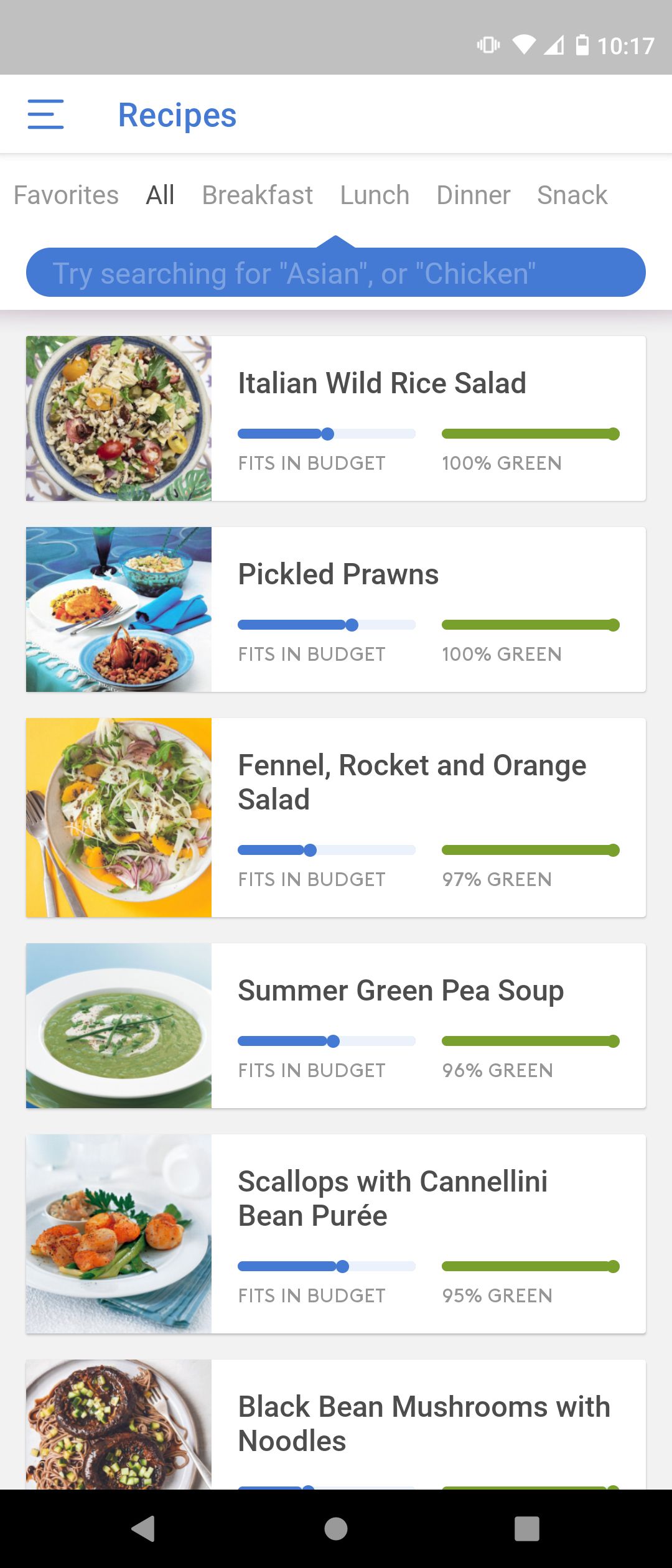Screenshot of a recipe page taken at 10:17 AM, featuring various types of meals sorted under multiple tabs: Favorites, All, Breakfast, Lunch, Dinner, and Snack. The screenshot is tagged under 'All' recipes. Listed recipes include:

1. **Italian Wild Rice** - Fits in budget, 100% green.
2. **Pickled Prawns** - Fits in budget, 100% green.
3. **Fennel Rocket and Orange Salad** - Fits in budget, 97% green.
4. **Summer Green Pea Soup** - Fits in budget, 96% green.
5. **Scallops with Cannellini Bean Puree** - Fits in budget, 95% green.
6. **Black Bean Mushrooms with Noodles** - Fits in budget, green-rated.

Each recipe is accompanied by a photo, showcasing what the dish looks like. The list appears to be organized in descending order of their 'green' rating.